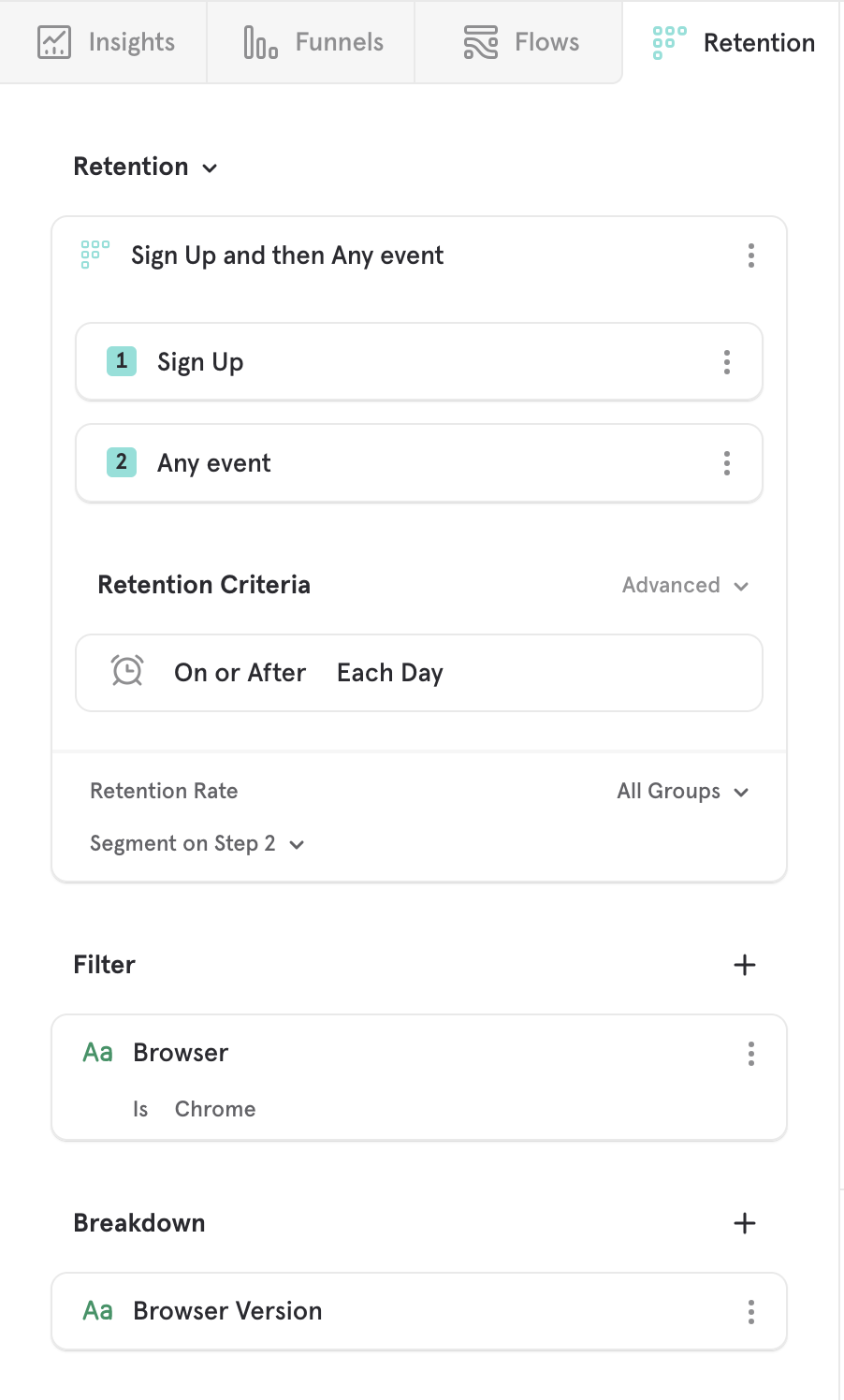The image depicts a user interface for analyzing website performance metrics, including sections for "Sites," "Funnels," "Flows," and "Retention." The "Retention" section is highlighted multiple times, suggesting its importance. A series of steps and data points are illustrated: 

1. "Sign Up" events followed by "Any Event," labeled sequentially as "1, 2, Any Event, 3, 6, 9 dots."
2. Retention criteria are accessible through an "Advanced" dropdown menu, indicating options such as "Alarm," "On or After," and "Each Day."
3. The "Retention Rate" is displayed for "All Groups," with an option to segment by "Step 2" available via another dropdown.
4. Filters can be applied using a "Filter Plus" button, marked by a capital "A" and a lowercase "a" in green.
5. Browser-specific data is segmented, showing distinctions for various browser versions alongside icons with three dots for additional options.

The background of the interface is mainly white, adding to its clarity and user-friendliness. However, parts of the interface background may appear green when showcasing particular details or dropdown menus.